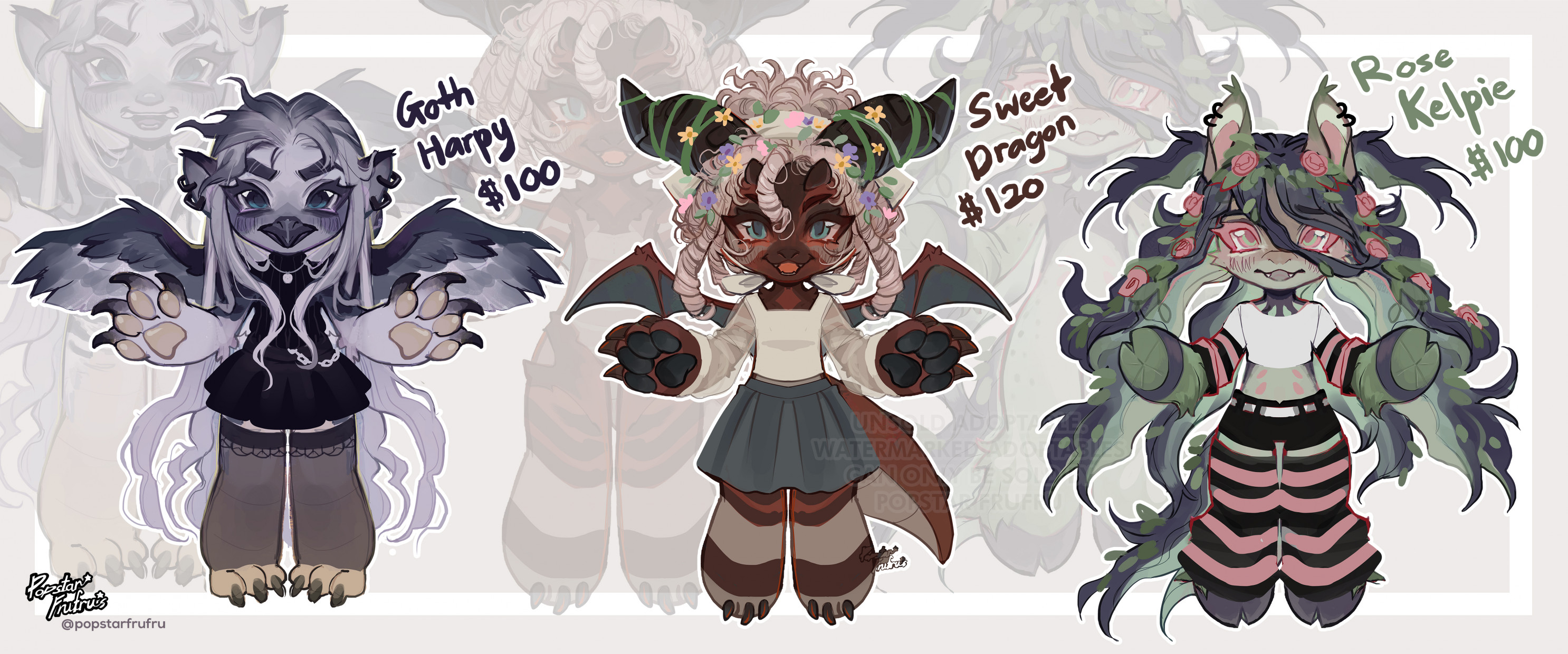This image showcases three cartoon-style fantasy dolls created by the artist PopstarBoopBoop, featuring colorful and fantastical designs. 

On the left, there's the "Goth Harpy" priced at $100, a dark blue and gray winged creature with noticeable claws and a gothic aesthetic. In the center, the "Sweet Dragon" is listed for $120 and is depicted with gray wings, a white tank top, and a gray skirt, giving it a unique and charming appearance. On the right, the "Rose Kelpie" is available for $100, with a vibrant pink and green color scheme reminiscent of a watermelon. Each of these characters is represented with distinct visual details and imaginative features, making them unique collector items for sale. The artist's contact, @popstarfrufru, is indicated on the lower left, likely pointing towards their Instagram handle for more information or to make a purchase.